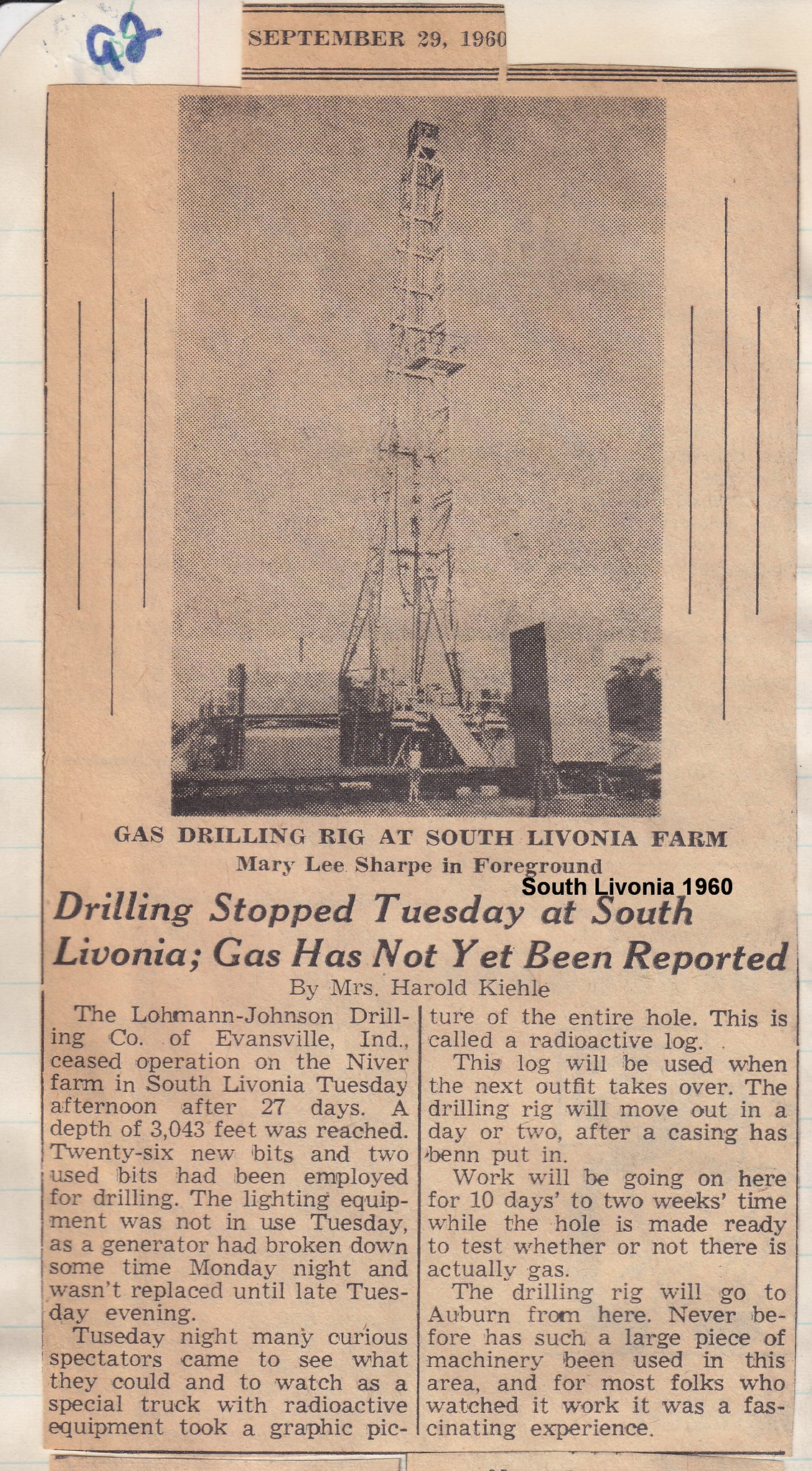This black and white image, likely a newspaper clipping, captures a towering gas drilling rig situated at South Livonia Farm. In the foreground, Mary Lee Sharp stands, grounding the scene amidst a couple of surrounding buildings and an expansive outdoor setting. The headline beneath the photograph boldly states, "Drilling Stopped Tuesday at South Livonia. Gas has not yet been reported." This article, penned by Mrs. Harold Kiley and dating back to 1960, details the halted drilling operations and notes the unconfirmed presence of gas. The aged, cream-toned paper forms the background, adding to the historical ambiance of the photograph and article. The image was likely taken during the day, optimizing natural light to emphasize the central drilling rig and its towering presence over the landscape.